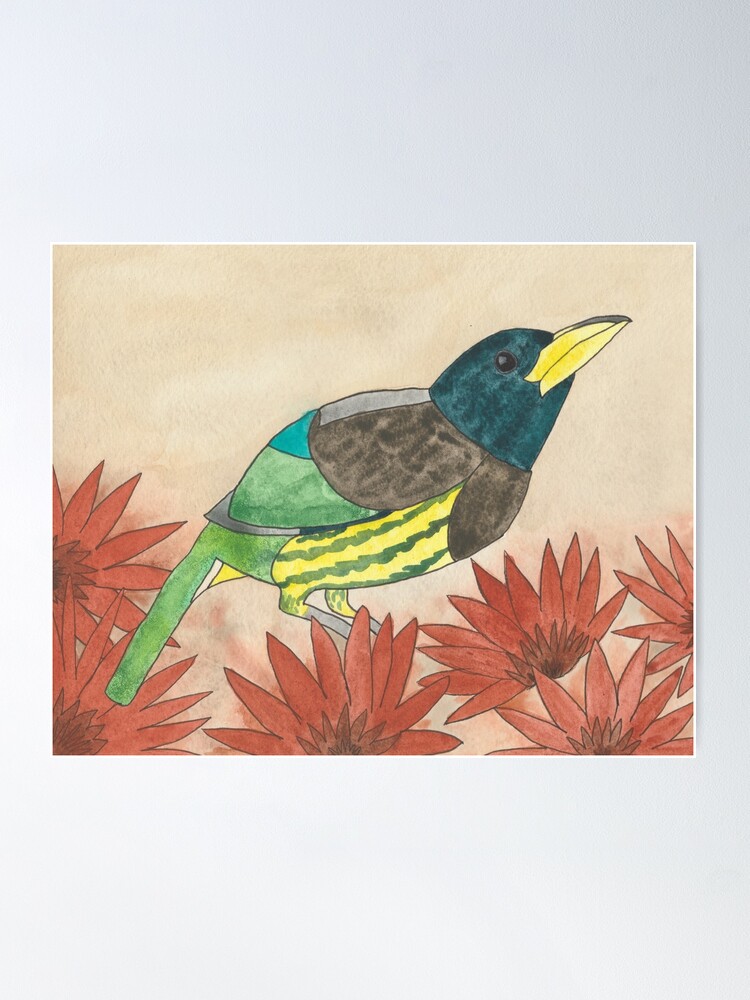This detailed artwork depicts a stylized bird positioned centrally among six spiky red flowers, set against a smudged beige background. The simplicity of the watercolor style and the thin black ink outlines lend the painting a unique charm. The bird stands on the bottommost flower with its gray legs. Its body features a bright yellow belly with dark brown swirling highlights, and a light green tail extending in a rectangular shape towards the bottom left. The bird’s upper wing area shows a combination of dark brown and light green, with a teal blue triangle accentuating the wing tip. Its head, a velvety bluish-green, features a glossy black eye and a large, curved, pointed yellow beak. The painting, mounted on a light gray to white wall, is highlighted by the contrast between the intricate details of the bird and flowers and the subtle background, emphasizing its delicate yet vibrant nature.